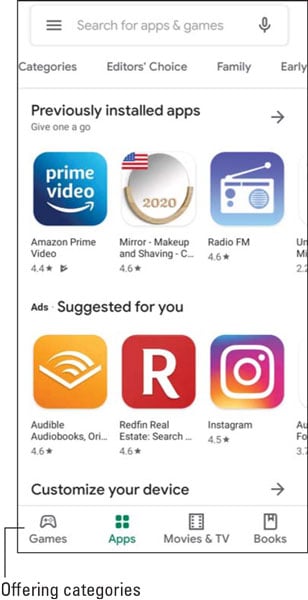The image appears to be a screenshot from a website featuring a search page for apps and games. 

At the top of the page, there is a search bar with three horizontal bars on the left, a gray text in the middle that reads "Search for apps and games," and a microphone icon on the right.

Below the search bar, the navigation menu contains the following categories in gray text: "Categories," "Editor's Choice," "Family," and an option labeled "Early" that is partially cut off by the image.

Beneath the navigation menu, in bold black lettering, it states "Previously installed apps," with a gray subtitle that reads "Give one a go." There is also an arrow pointing to the right next to this subtitle.

The section below lists previously installed apps:
1. The first app is Amazon Prime Video, represented by a blue box logo with the white text "Prime Video" and the recognizable Amazon smile logo. Beneath this, it says "Amazon Prime Video."
2. To the right of Amazon Prime Video, there's an icon resembling a mirror with "2020" in gold beneath it. The text below reads "Mirror - Makeup and Shaving."
3. Next, there's a blue box with a white radio outline inside. The text below this icon says "Radio FM" in black.

Following this section, in black text, it says "Suggested for you:"
1. The first suggestion is a gold box with a white outline of a book and three lines representing text between the pages. Below this, it says "Audible Audiobooks."
2. Next to Audible, there's a red box with a white "R" and the text "Redfin Real Estate Search" below it.
3. Lastly, there is a rainbow-colored box transitioning from blue at the top to orange at the bottom, featuring a white camera lens icon. The text below reads "Instagram."

The final section of the image contains black text that says "Customize your device."